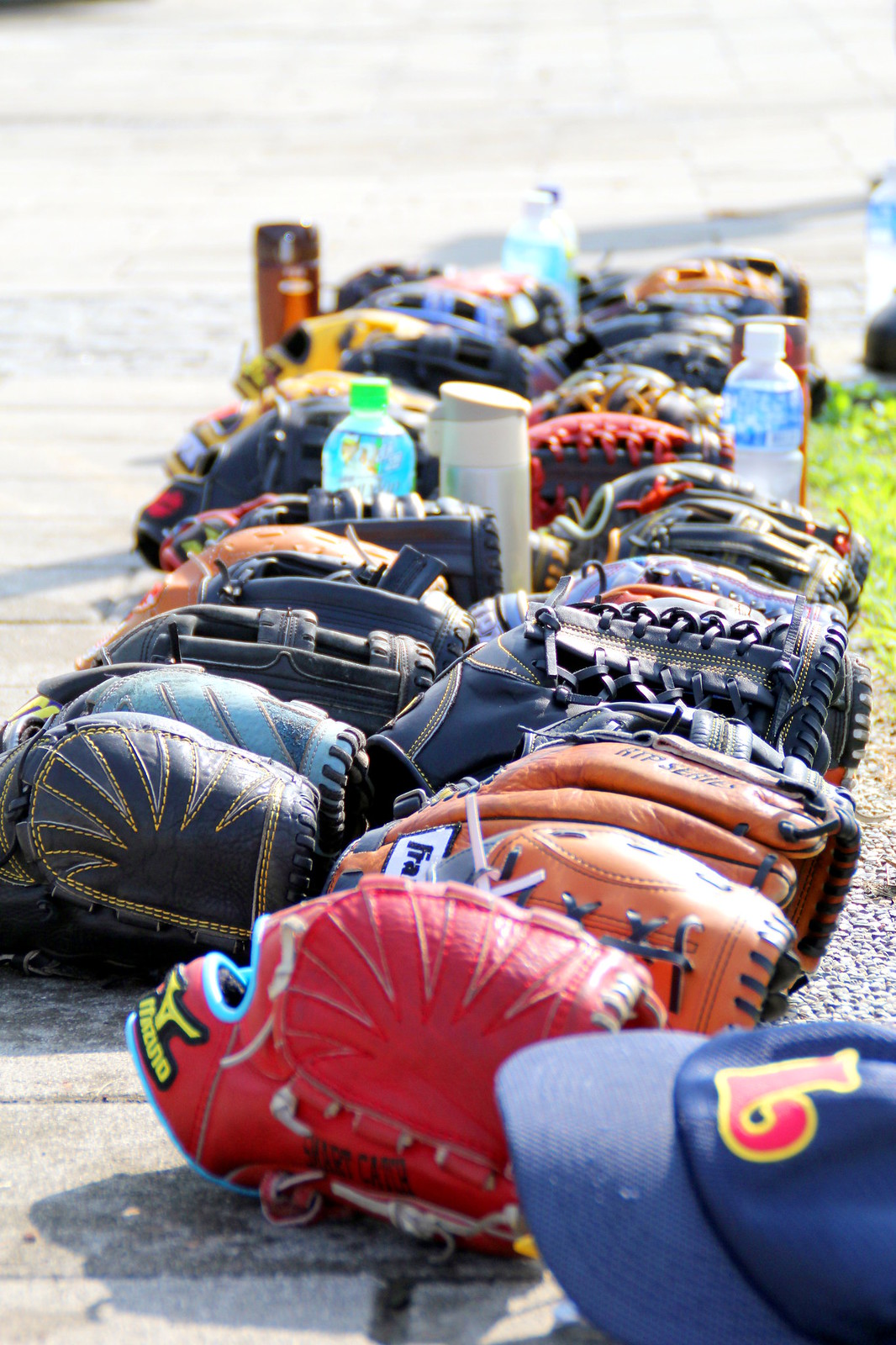This vibrant outdoor image showcases an array of baseball gloves meticulously lined up in two neat rows on interlocking brick pavement, next to a small patch of grass. The gloves, all with their interiors facing down, exhibit a striking variety of colors and designs, including red, green, orange, black, blue, brown, and tan. Amidst the gloves is a standout dark blue baseball cap adorned with a red letter 'B', and a bright red glove featuring a yellow letter 'K'. Interspersed amongst the gloves are a number of water bottles, mostly clear with labels, with a noticeable red bottle at one end. The scene is bathed in sunlight, suggesting a bright and possibly blistering day, as the sun reflects off the pavement. The image captures a moment of stillness and order among the used, yet carefully arranged, baseball gear.